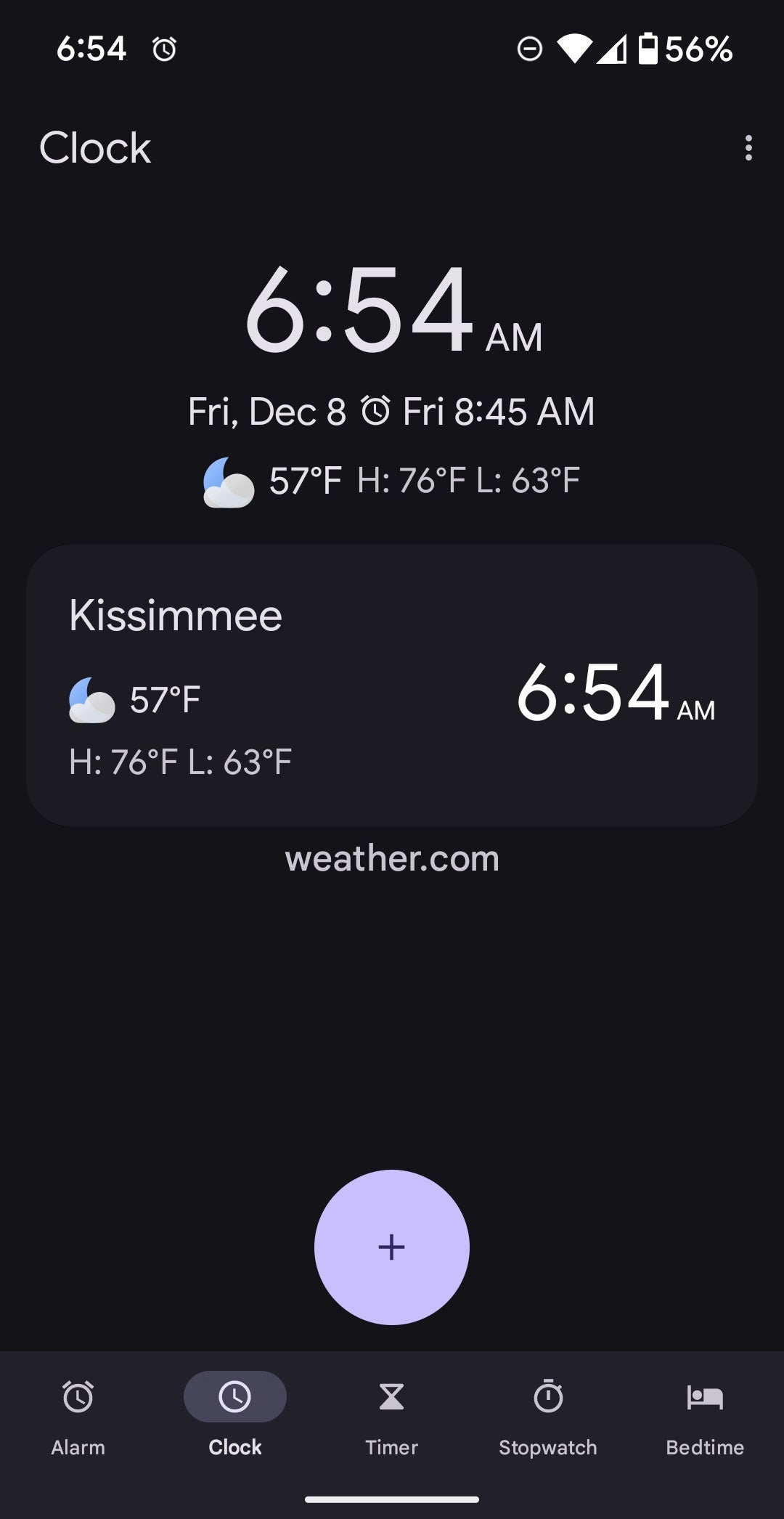This image is a detailed screenshot of a smartphone's lock screen. At the top left, the time is displayed as 6:54 AM. Adjacent to the time on the upper right, various icons including an alarm clock, Wi-Fi signal, cellular reception, and a battery indicator show the battery life at 56%. Directly beneath the time, the word "Clock" is written on the left side.

Centered at the top, the bold, large numbers display the current time as 6:54 AM again, and below it, the date is indicated as "Friday, December 8." Further down, there is an alarm icon next to "Friday, 8:45 AM" indicating a scheduled alarm time.

The weather information is also present, featuring an icon of a moon with a cloud, suggesting nighttime or early morning conditions, and a current temperature of 57°F. Additionally, it provides the day's high temperature as 76°F (H: 76°F) and the low as 63°F (L: 63°F). An "Add" symbol is visible at the bottom of the screen, indicating an option to add more widgets or features. This comprehensive lock screen provides the user with crucial time, date, alarm, battery, and weather details at a glance.